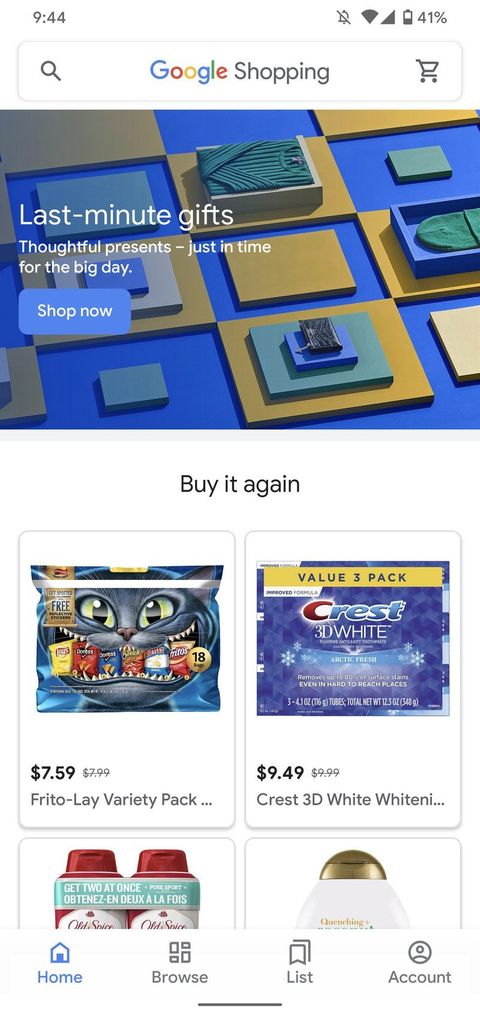The image depicts a screenshot of a mobile device. At the top left corner, the time is displayed as 9:44. On the top right, several status icons are visible, including a mute icon, a Wi-Fi signal icon showing full bars, a network signal icon also showing full bars, and a battery level indicator reading 1% plus. 

Below the status bar, the screen showcases the Google Shopping interface. Prominently displayed text reads "Last Minute Gifts: Thoughtful presents just in time for the big day. Shop Now." Further down, the interface suggests popular items, featuring products such as a Frito-Lay Variety Pack priced at $7.59 and Crest 3D White toothpaste priced at $9.49.

At the bottom of the screen, navigation icons for major categories are visible: Home, Browse, List, and Account. Additionally, a shopping cart icon is positioned to the right, with a search magnifying glass to the left.